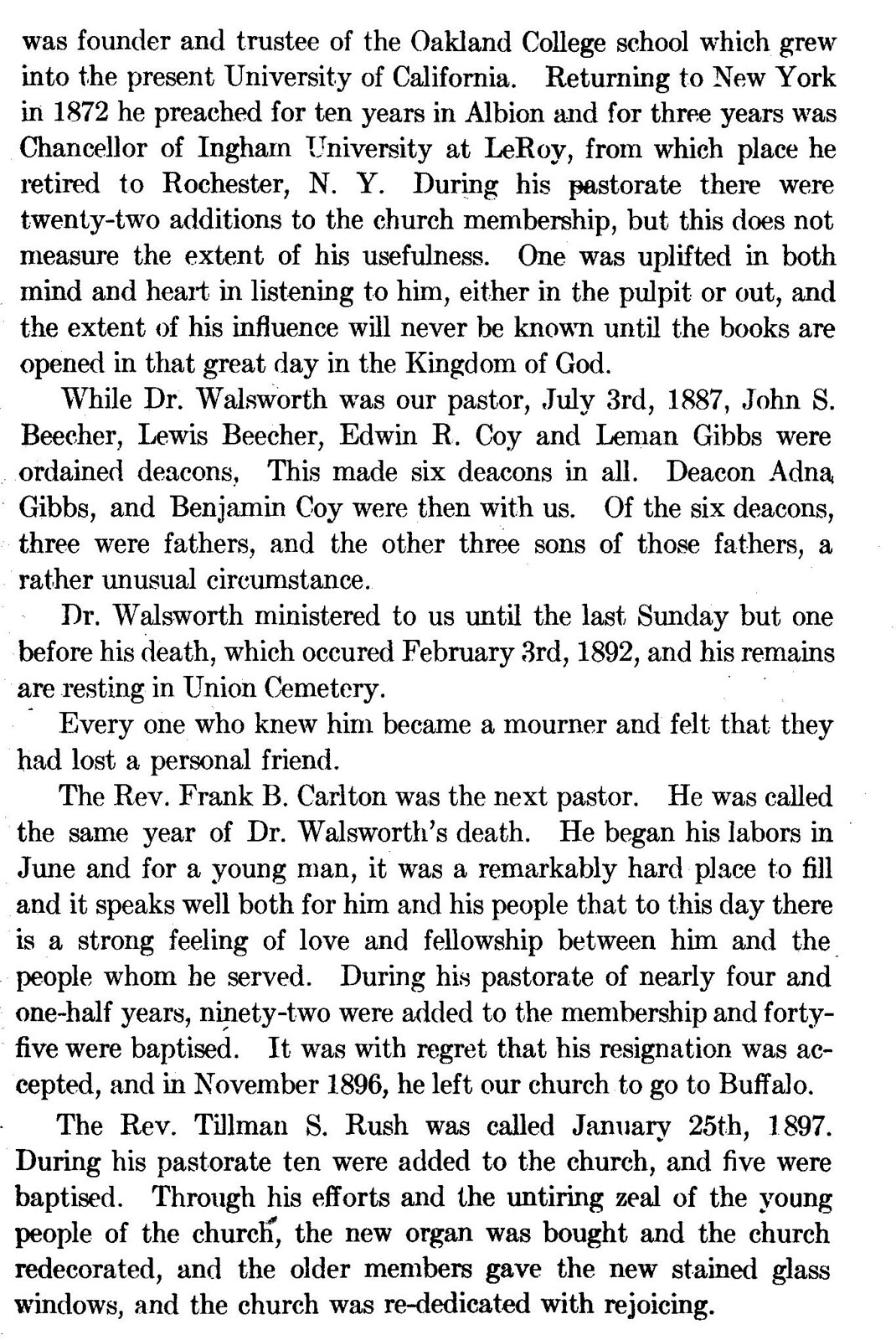The image depicts a scanned page from an old book or article with a white background and long columns of small, black text. The text details the life and career of Dr. Walsworth, highlighting his significant contributions. It begins with his role as the founder and trustee of the Oakland College School, which later became the University of California. After returning to New York in 1872, he preached for a decade in Albion and served as Chancellor of Ingham University at LaRoy for three years before retiring to Rochester, NY. The document also notes that Dr. Walsworth ministered until shortly before his death on February 3rd, 1892, with his remains resting in Union Cemetery. Additionally, it praises his lasting influence on church membership and the upliftment of minds and hearts through his sermons, acknowledging his profound, though immeasurable, impact.